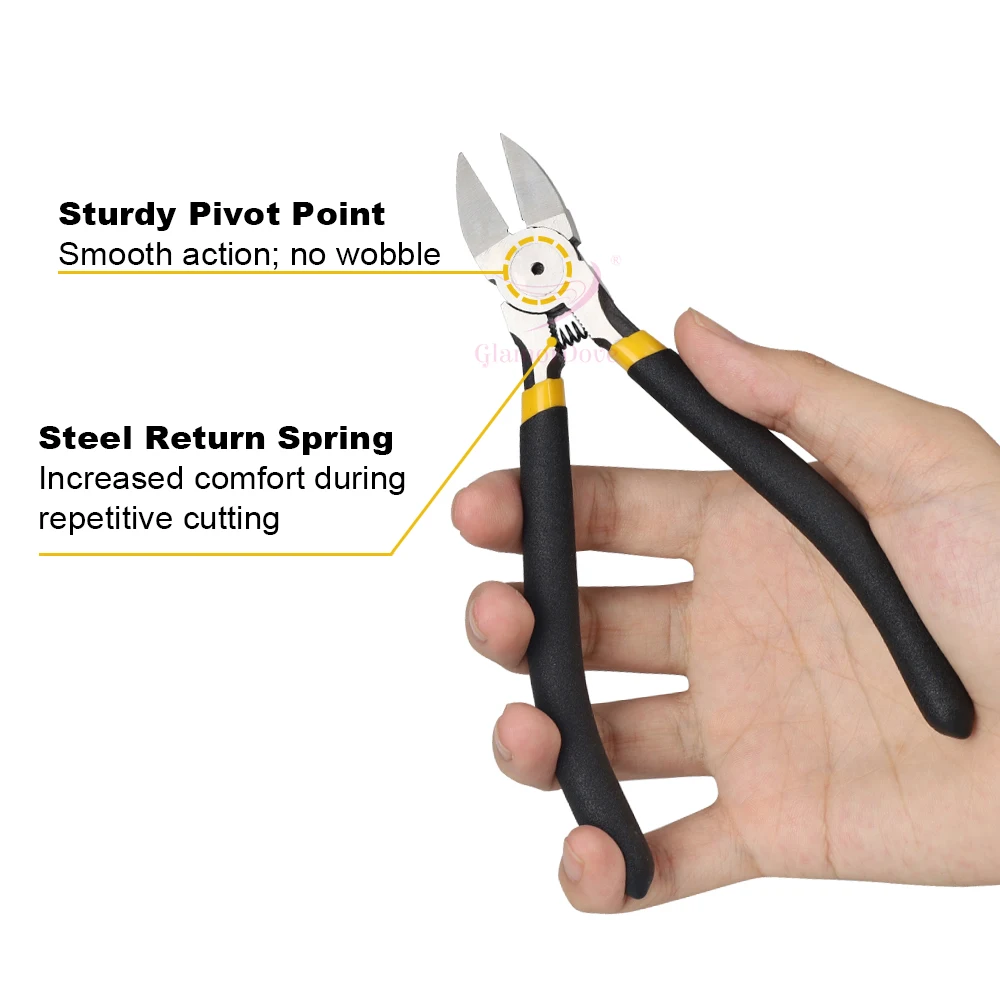The image showcases an advertisement with a white background and no border, featuring a pair of pointed, silver wire cutters or needle-nose pliers. The pliers have a black handle with yellow trim at the tips and are held diagonally by a hand, with four fingers wrapped around one handle and the thumb on the other. A black spring is positioned between the handles, enhancing comfort for repetitive cutting. Adjacent to the pliers, labels with yellow arrows provide product details. One arrow points to the center of the tool, highlighting its "Sturdy pivot point, smooth action, no wobble." Another arrow points to the spring, noting "Steel return spring, increased comfort during repetitive cutting."